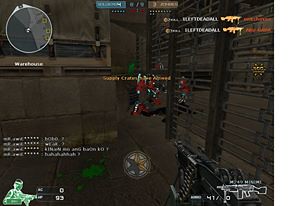This screenshot, likely from a computer or console video game, features a complex and dynamic scene. The image is set in a landscape orientation and is slightly more rectangular than square. The background consists of a concrete or brownish terrain, with a barrier formed by a series of loop-like metal pieces on the left, resembling a fence.

In the forefront, a character is wielding a large black firearm, with a visible ammunition clip encircling it. To the left of the screen, there is a section of white text, possibly indicating game stats or objectives. The bottom left corner displays an icon of a person holding a gun, which is green but appears to be depleting in color like a health or stamina meter.

At the top of the screen, a compass-like map aids in navigation, while the center of the screen is filled with red-clad characters engaged in combat, suggesting a chaotic battle scene. The top right corner features two orange gun icons accompanied by white text, possibly showing weapon status or ammunition count.